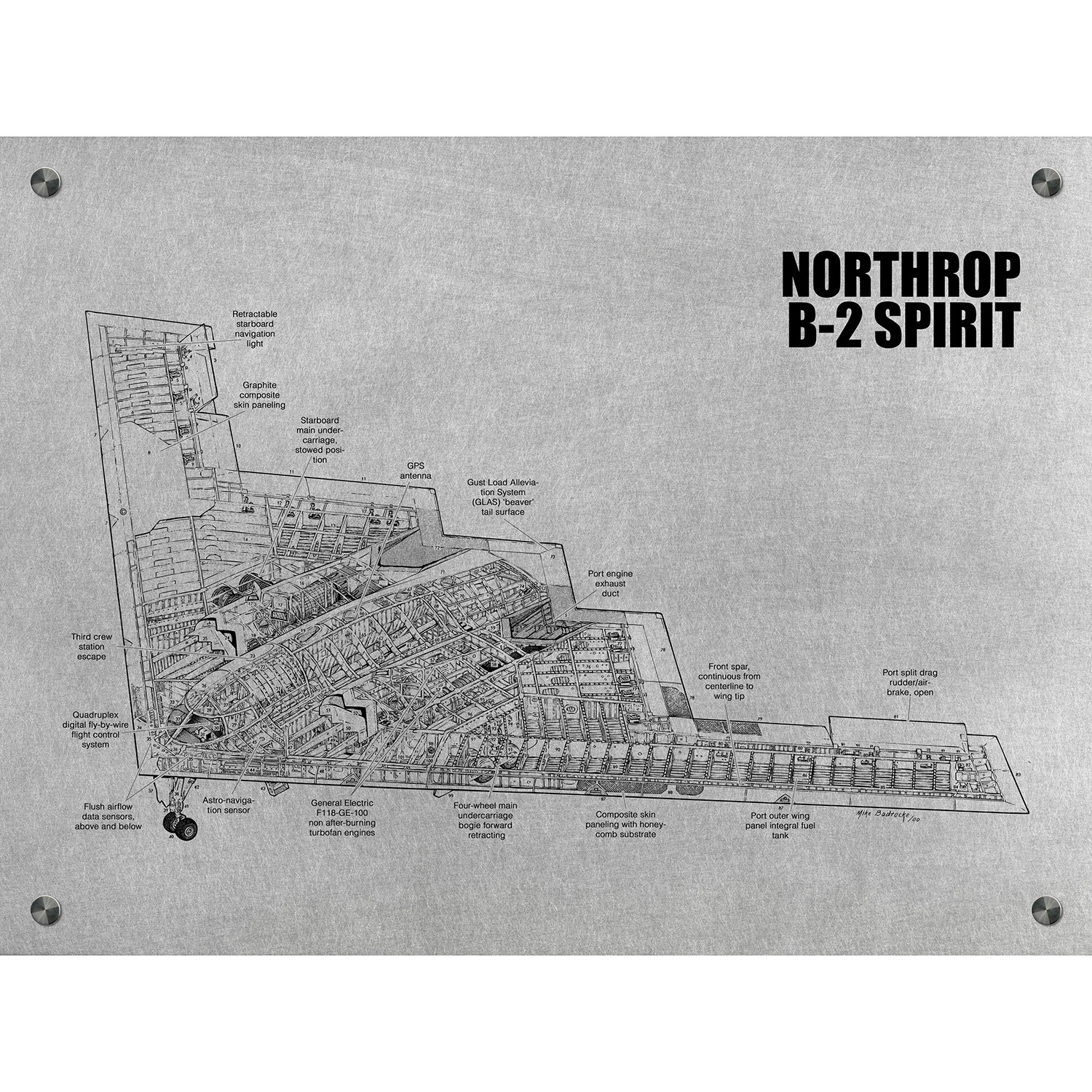This is a highly detailed black-and-white schematic of the Northrop B-2 Spirit, commonly known as the Stealth Bomber, depicted almost like an x-ray image. The diagram showcases the intricate inner workings of the aircraft, including components such as the flaps, cockpit, retractable starboard navigation light, graphite composite skin paneling, starboard main undercarriage, GPS antenna, port engine exhaust duct, and the front spar extending to the wingtip. Various technical labels annotate these parts, providing specific explanations and highlighting areas like crew stations and airflow systems. The image, which might be pinned to a wall, appears to be printed on a metallic sheet or a gray piece of paper and features the title "Northrop B-2 Spirit" at the top right corner. Its detailed and architectural design suggests it functions as a blueprint, perhaps intended for reference in a technical manual or display.